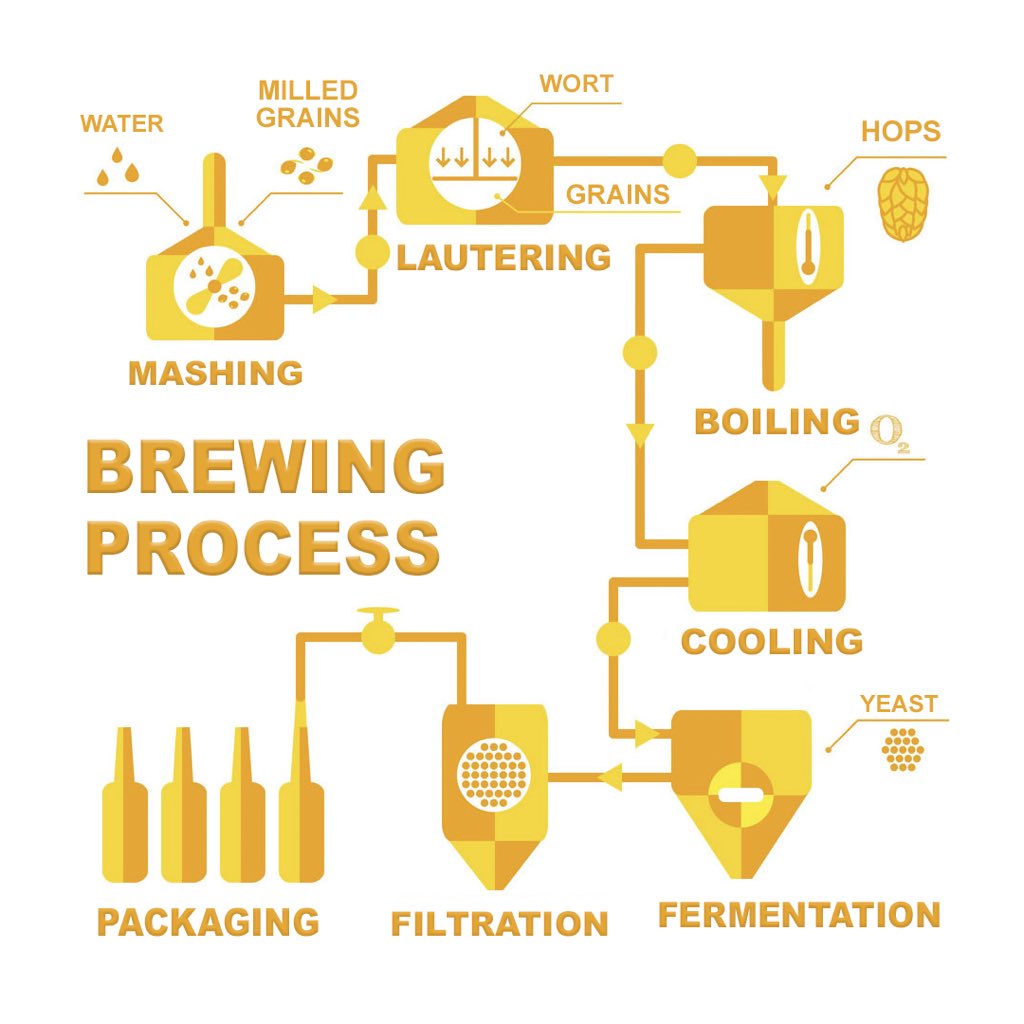The image is a detailed diagram of the brewing process, vividly illustrated in varying shades of yellow on a white background. Starting from the top left, the process begins with a machine labeled "Mashing," where water and milled grains are combined. An arrow leads to the right, pointing to the next stage, "Lautering," where the wort is separated from the grains. Moving further right, the diagram shows the "Boiling" stage, followed by "Cooling." The process then transitions downward, illustrating "Fermentation" where yeast is added to the mix. Further steps include "Filtration" and finally "Packaging," where the finished product is bottled for distribution. The entire flowchart runs from the top left, across to the right, and then down towards the bottom of the image. On the left side, the words "Brewing Process" are prominently displayed in yellow, detailing each crucial stage in beer production.